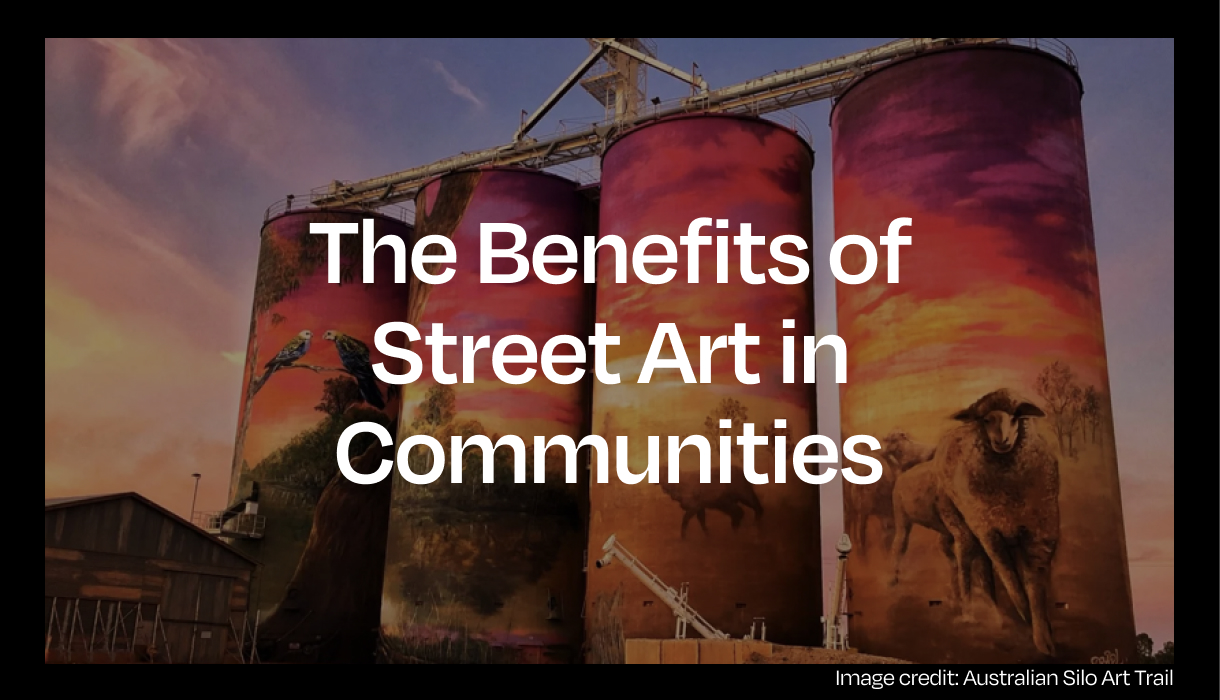This is a color photograph of an advertisement poster featuring an image of four large cylindrical silos. These silos are seamlessly painted to create a single, continuous mural illustrating a picturesque rural scene. The top of the mural depicts a serene dusk or dawn sky with rich shades of purples, yellows, reds, oranges, and blues, interspersed with pink, orange, and white clouds. There are birds perched on branches to the left, while the right silo showcases forward-facing sheep set against green pastures dotted with grasses and rolling hills. A small, old wooden barn is visible at the bottom left corner. White text overlays the image, boldly stating: "The Benefits of Street Art in Communities." The bottom right corner credits the "Australian Silo Art Trail" for the image.